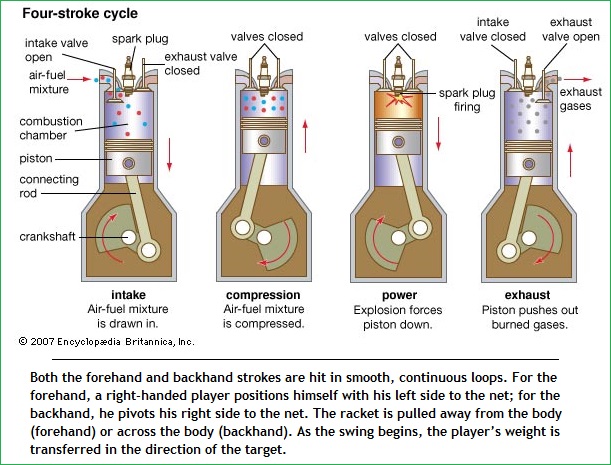The image titled "Four-Stroke Cycle" from the 2007 Encyclopedia Britannica, Inc. showcases a detailed diagram of the internal processes within an engine, emphasizing the four main stages: Intake, Compression, Power, and Exhaust. 

Each of the four cylindrical illustrations from left to right demonstrates distinct stages: 

1. **Intake (leftmost)**: Marked at the top with "spark plug" and labeled "exhaust valve closed," this stage shows the air-fuel mixture being drawn into the combustion chamber via downward-facing red arrows, with accompanying labels such as air-fuel mixture, combustion chamber, piston, connecting rod, and crankshaft.

2. **Compression** (second from the left): Highlighted by closed valves and an upward red arrow, this stage depicts the compression of the air-fuel mixture within the chamber.

3. **Power** (third from the left): This illustrates the explosion forcing the piston down as the spark plug fires, shown by a downward red arrow and the only orange-hued area indicating the explosion's intensity.

4. **Exhaust** (rightmost): Here, the piston expels burnt gases through the open exhaust valve, accompanied by red arrows pointing up and to the right, and labels indicating exhaust gases.

The diagram is ensconced within a thin green outline on a white background with the title "Four-Stroke Cycle" at the upper left. A separate section at the bottom contains a seemingly unrelated paragraph about tennis strokes, printed in black text across four and a half lines, describing the movements and weight transfer of a player executing forehand and backhand strokes.

Overall, the image combines technical illustrations with detailed annotations to explain the internal combustion engine's four-stroke cycle, visually separating it from the unrelated text about tennis.